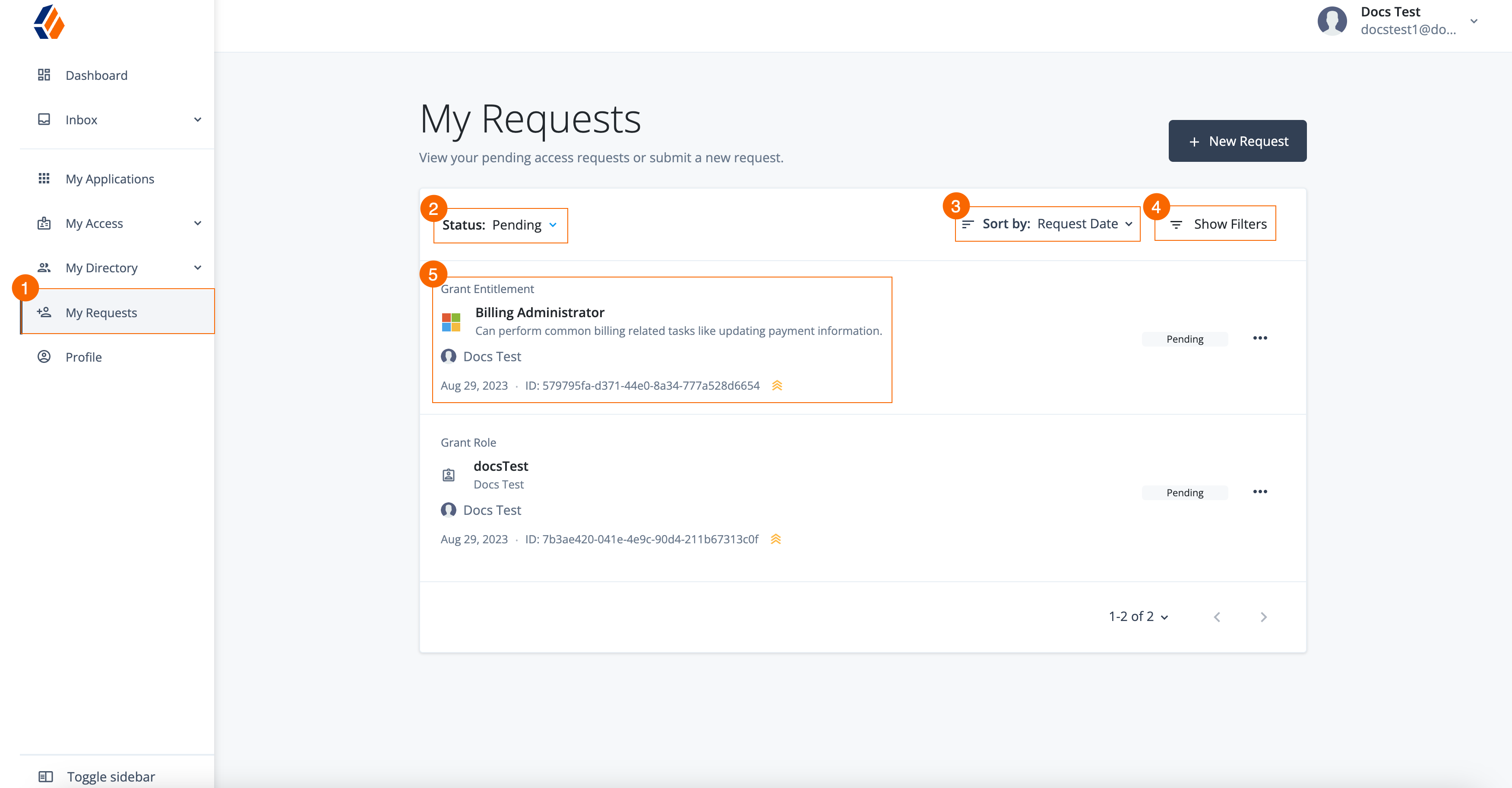This image falls under the "Websites" category and shows a user interface with a distinct layout. In the top left corner, there's a unique square icon featuring blue edges and an orange face. Down the left side of the interface, a vertical navigation menu lists options: Dashboard, Inbox, My Applications, My Account, My Directory, My Requests, and Profile. The "My Requests" option is highlighted and displays a notification badge with the number 1.

The "My Requests" section is open, revealing the text "View your pending access requests or submit new requests." The user interface appears to be guiding someone through the steps to accomplish a task, labeled sequentially:

1. A box labeled "Status Pending" is marked with the number 2, accompanied by drop-down menus.
2. A box labeled "Sort by Request Date" is identified with the number 3.
3. The number 4 designates a section labeled "Show Filters."
4. The number 5 corresponds to a section labeled "Grant Entitlement."

In the "Grant Entitlement" section, identified by a window symbol, there's a title "Billing Administrator," with a description: "Can perform common billing-related tasks like updating payment information." Below this, another label reads "Docs Test."

This detailed caption succinctly describes the visual elements and organized steps presented within the user interface.